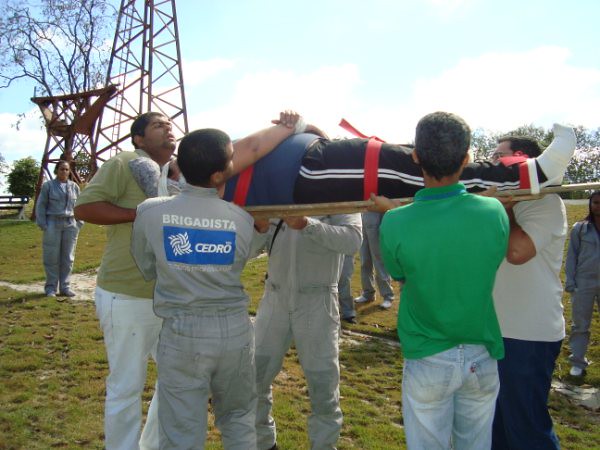In a grassy field under a hazy, cloudy sky, a group of five men carry a person secured to a homemade stretcher, which is held at shoulder height. The stretcher, fashioned out of simple materials, features red straps that firmly secure the individual, who is dressed in a blue shirt and black running pants with a white stripe down the side. The person on the stretcher has their hands crossed over their stomach and is wearing white socks, visible on one foot. Among the men carrying the stretcher, one on the right has black hair, a black back of his head, and is wearing a green collared shirt with light blue jeans. Next to him, another man wears a long-sleeved gray shirt with the words "Brigadasta Cedro" in white text and a blue rectangle underneath. In the background, bystanders watch the scene unfold, which appears to be a training exercise or an emergency drill rather than a real medical emergency. Looming in the distance is a tall, rusted radio tower made of metal poles that narrows as it ascends. Surrounding the group, the uneven grass terrain is dotted with bulges and patches, reflecting the outdoor, daytime setting.